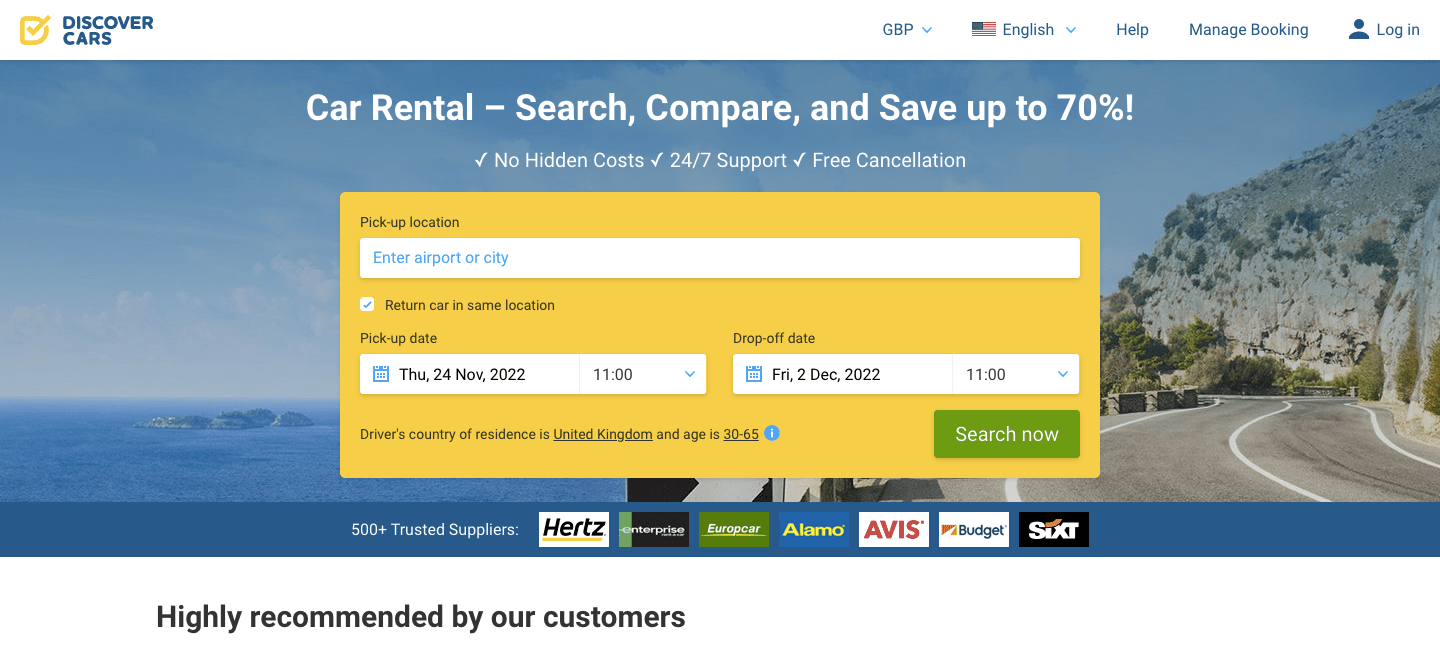In the upper left corner of the image, there is a white strip running across the top. Starting from the middle and extending to the right, the text "GBP" appears alongside a drop-down menu, followed by "English" accompanied by an American flag and another drop-down menu. Further along, there are icons for help, manage booking, and a person icon with the label "Login" next to it.

Below this header is a photograph featuring a road on the right side bordered by cliffs, and water on the left side. Overlaying this image, text reads "Car Rental - Search, Compare, and Save up to 70%." Additional text below mentions "No Hidden Costs," "24/7 Support," and "Free Cancellation."

A yellow rectangle bears the label "Pick-up Location" with an adjacent data field in blue font stating, "Enter airport or city." Below, the text "Return car to the same location" is checked off. The "Pick-up Date" is listed as "Thursday, 24 November 2022, 11 AM" with an associated drop-down menu. Next to it, "Drop-off Date" is stated as "Friday, 2 December 2022, 11 AM," again with a corresponding drop-down menu.

Further down, there is a section labeled "Driver's country of residence" displaying "United Kingdom," which is underlined, and "Age 30 to 65," also underlined. To the right side, there is a blue circle with a white information 'i' in it, and next to it is a "Search Now" button.